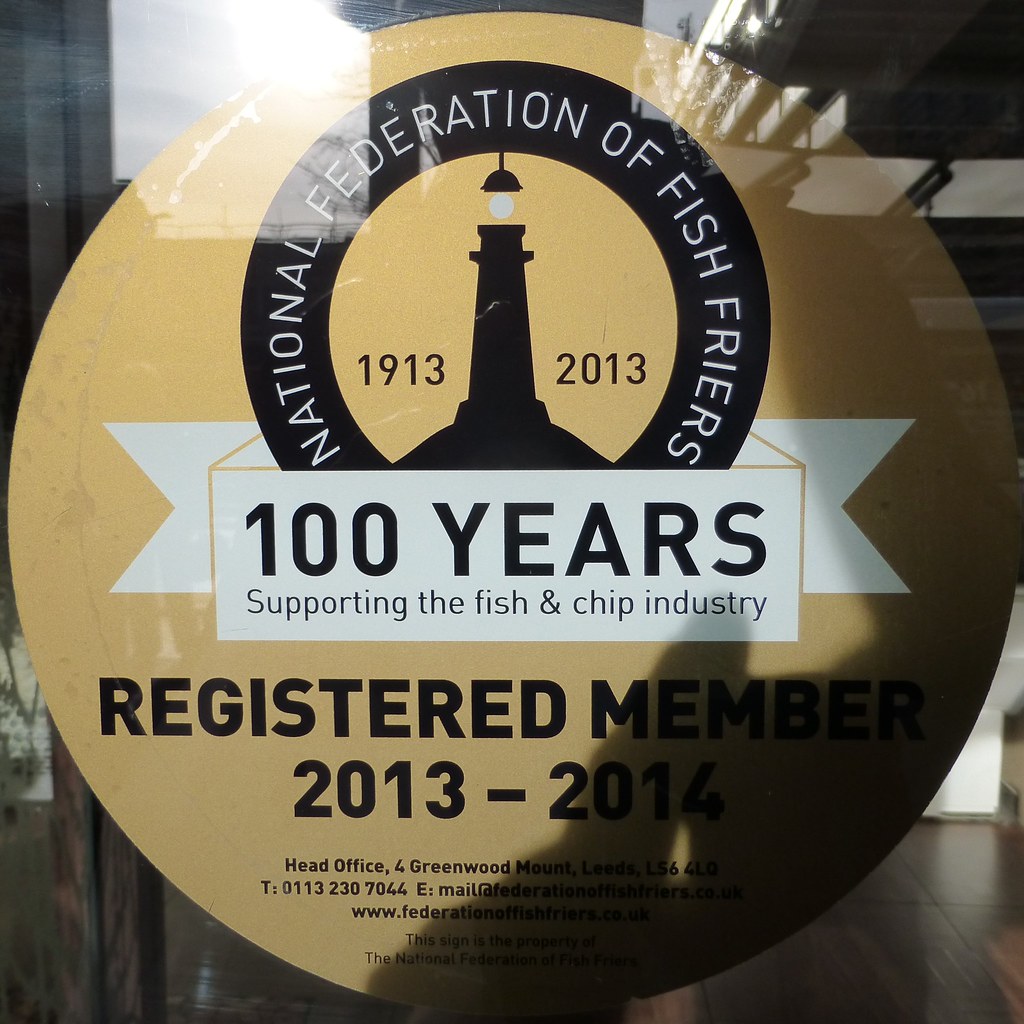The image is of a glass pane, and through it, one can see a sticker with a design in a circular shape. The circle has a gold background and prominently features a black lighthouse in the center. Encircling the lighthouse is a black border with white text that reads, "National Federation of Fish Fryers." Inside the circle, flanking the lighthouse, the dates "1913" and "2013" are displayed. Below this, a white banner with black text states, "100 years supporting the fish and chip industry." Further down, in bold black text, it says, "Registered Member 2013-2014." Additional smaller text provides the head office address: Greenwood Mount, Leeds, LS12 4LQ, and contact details, including a telephone number (0113 230 7044) and an email address (mail@federationoffishfryers.co.uk). Also mentioned is the website, www.federationoffishfryers.co.uk, along with a notice in small print stating, "This sign is the property of the National Federation of Fish Fryers." There is a reflection on the glass pane, hinting at shadows outside, and some brown tile flooring is visible at the top of the image.